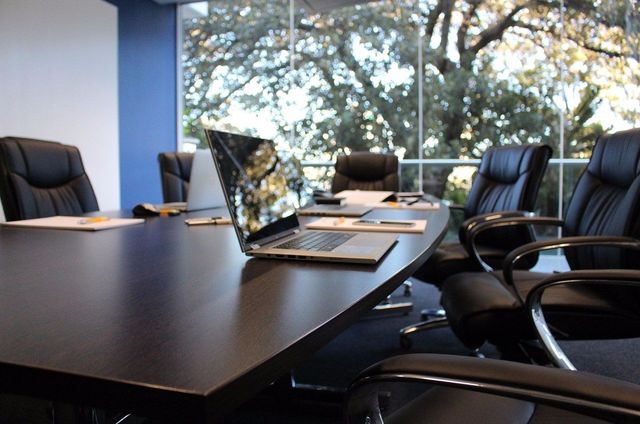The photograph captures a detailed view of a professional boardroom setting. At the center, a slightly curved, dark brown wooden table spans almost the entire frame. This table is surrounded by six executive chairs, each featuring black leather upholstery and stainless steel armrests with black padding on top. On the table, which is rectangular with curved edges, are two laptops positioned near the middle, accompanied by paper notepads and pens arranged neatly. The background showcases a large window with a sleek, skinny frame that allows an out-of-focus view of a lush green tree and sky. To the left of the window, there is a blue pillar adjacent to a white wall, adding a touch of color contrast to the overall muted palette of the room. The scene conveys an air of readiness and professionalism, with all seats empty and waiting for occupants.